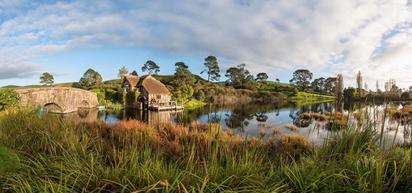The image showcases a serene and picturesque landscape featuring a tranquil, reflective body of water centrally located amidst tall, lush green grass interspersed with patches of brown and beige. In the immediate foreground, the vibrant grass gives way to a clear, mirror-like pond or lake which perfectly reflects the surrounding scenery, including the blue sky and white clouds above. To the left, a small, beige-colored stone bridge with two arches spans the water, accompanied by a small tree growing on its side.

Just beyond the bridge, on the left side of the landscape, stands a charming single-story house with a triangular roof of brownish color and lighter brown walls. The house includes an attic-like attachment, adding a quaint character to the scene. Behind the house, a gentle hill is dotted with trees, extending the lush green and natural feel even further. The image is bathed in bright, clear lighting, enhancing the overall vividness and detail of the landscape.